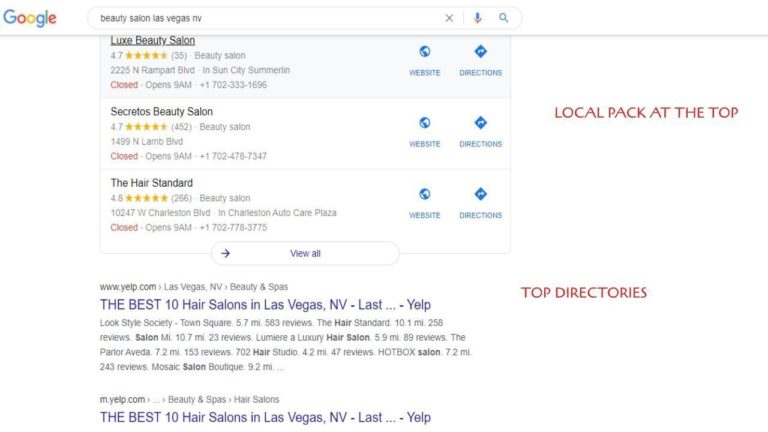The image shows a Google search results page. At the top left corner, the Google logo is visible. Below it, a white search bar contains the query "Beauty Salon Las Vegas Envy" in black text. The search results displayed are as follows:

1. **Lux Beauty Salon**:
   - Rating: 4.7 stars (35 reviews)
   - Address: 2225 North Rampart Boulevard, Sun City, Summerton
   - Status: "Closed" highlighted in red, "Opens 9 a.m."
   - Phone Number: +1 702-333-1696

2. **Secretos Beauty Salon**:
   - Rating: 4.7 stars (452 reviews)
   - Address: 2225 North Rampart Boulevard
   - Status: "Closed" highlighted in red, "Opens 9 a.m."
   - Phone Number: +1 702-247-8734

3. **The Hair Standard**:
   - Rating: 4.8 stars (266 reviews)
   - Address: 10247 West Charleston Boulevard, Charleston, Auto Care Plaza
   - Status: "Closed" highlighted in red, "Opens 9 a.m."
   - Phone Number: +1 702-776-3775

There is also a white oval button with purple text that says "Review All". Below the search results, a link to Yelp is visible with the text "The Best Hair Salons in Las Vegas, NV - Yelp".